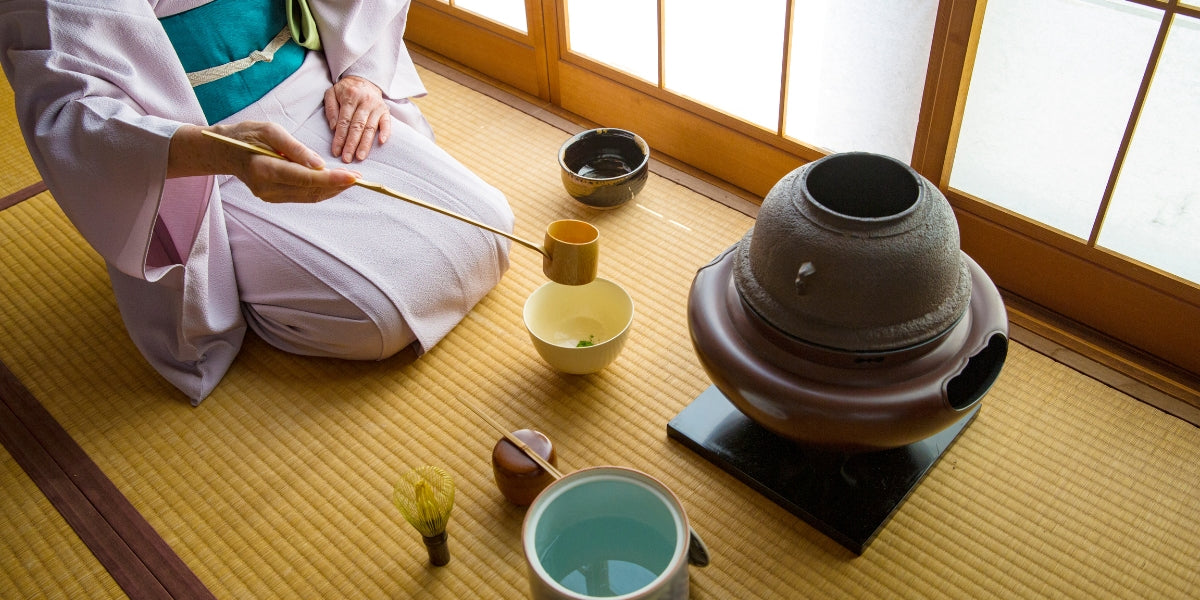This full-color photograph, captured in natural light, showcases a traditional Japanese tea service in a horizontally rectangular, landscape orientation. The setting reveals an indoor scene with a beige wooden frame and white translucent paper panels of a shoji screen in the background.

The central figure, a female, appears on the left side of the image, wearing a light pink kimono adorned with a pink apron and a wide turquoise tie around her waist. She is kneeling forward on a woven yellow straw mat, her legs tucked neatly beneath her. Her left hand rests on her hip while her right hand holds a long-handled wooden ladle with a beige cup, poised over a small yellow bowl as if pouring into it.

The scene includes an array of bowls and utensils: a small brown bowl situated just above the yellow bowl, and a larger pot with water positioned below, accompanied by additional utensils. A tall, oversized brown urn, with a rounded shape and set on a square black platform, occupies the right center of the image, partially visible from the top. Complementing these elements, various bowls in hues of brown, blue, and yellow are scattered around.

The photograph adheres to a representational realism style, capturing the intricate details and serene ambiance of the tea service ceremony.